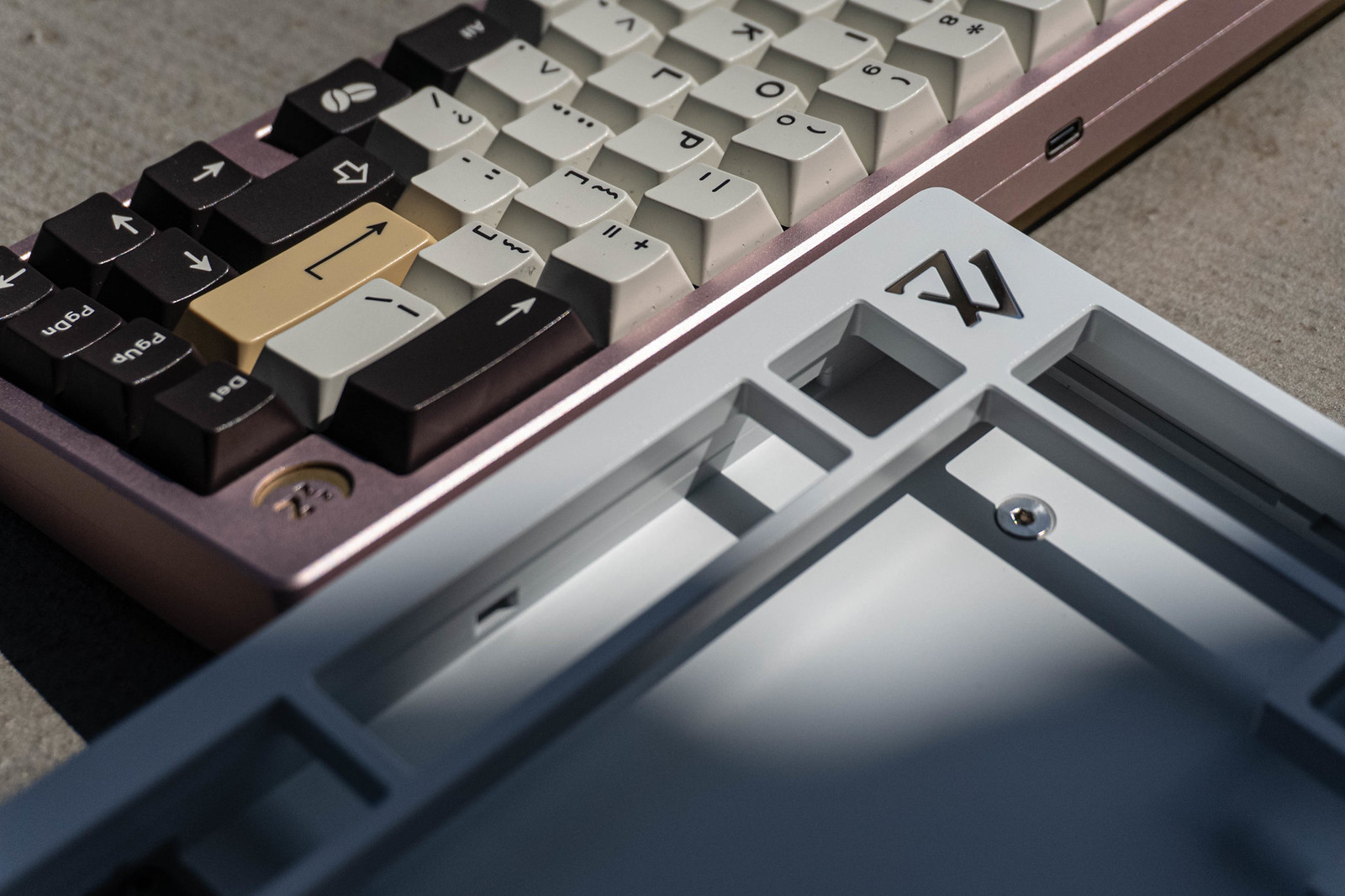The image features a uniquely designed keyboard, prominently positioned on an off-white surface, with a gray plastic frame in front of it. The keyboard itself has a silver frame and a mix of off-white, black, and a distinctive tan enter key. Notably, one key has the unusual symbol of two coffee beans. The control keys are off-white, with the backspace and arrow keys being black. The enter key stands out with its ivory color. The surrounding gray plastic piece features a logo resembling two carved triangles or a possible "7V" cutout. The overall image is slightly dark, adding to the enigmatic nature of the scene, as the exact purpose of the gray frame remains uncertain.